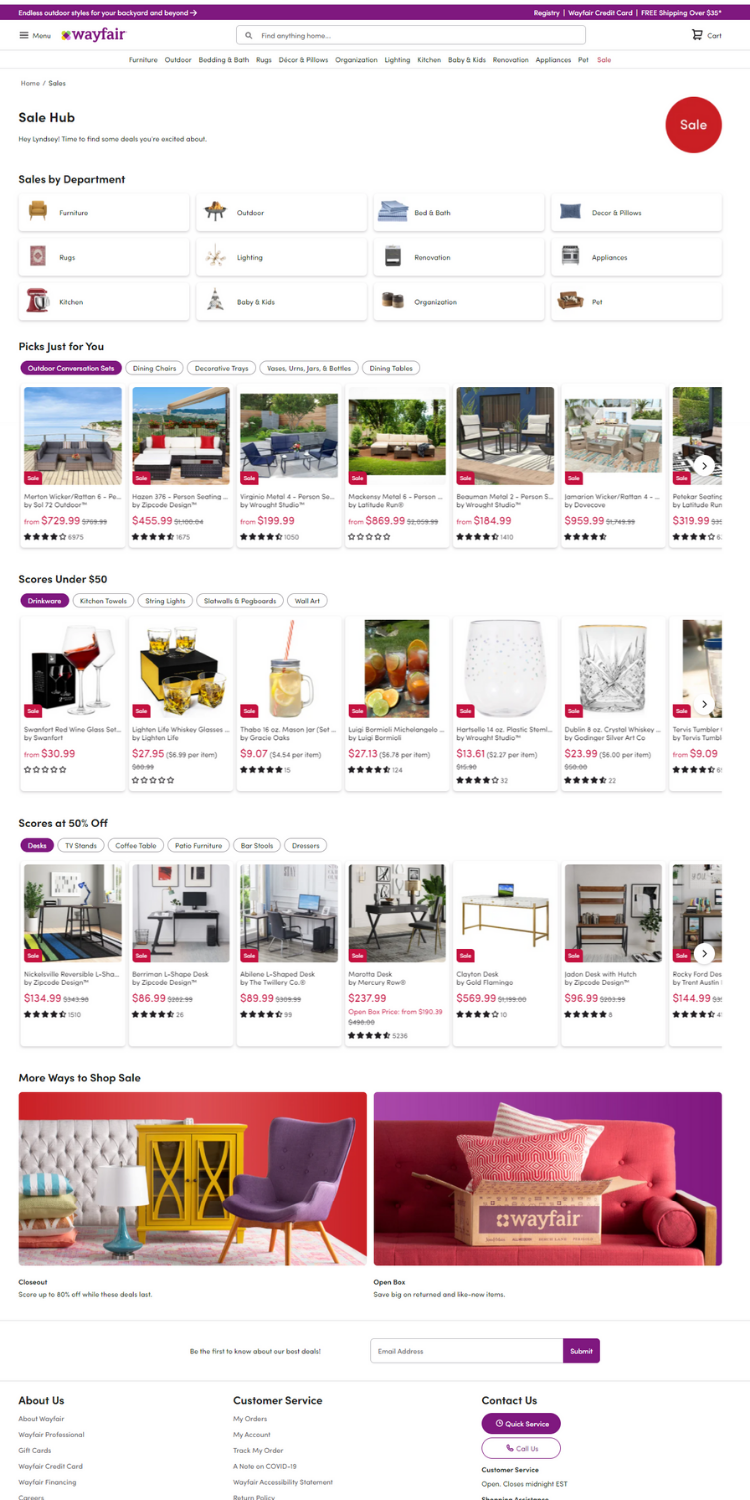The image is a screenshot of the Wayfair.com homepage. At the very top, you can see the Wayfair logo in purple, accompanied by an icon. Prominently displayed is a banner that reads "Endless outdoor styles for your backyard and beyond." A section labeled "Sale Hub" follows, with a friendly message saying, "Hi, Lindsay! Time to find some deals you're excited about." At the far right of this area is a red circle with the word "SALE" in bold white letters.

Scrolling down, the image showcases the "Sales by Department" section, which is organized into three rows, each containing four clickable buttons. In the first row, the categories are Furniture, Outdoor, Bed & Bath, and Décor & Pillows. The second row lists Rugs, Lighting, Renovation, and Appliances. The third row includes Kitchen, Baby & Kids, Organization, and Pet.

Further down, there are various curated sections like "Picks Just for You," "Scores under $50," "Scores at 50% off," and "More Ways to Shop and Save." The image finally shows the footer of the website, which contains additional navigation and informational links.